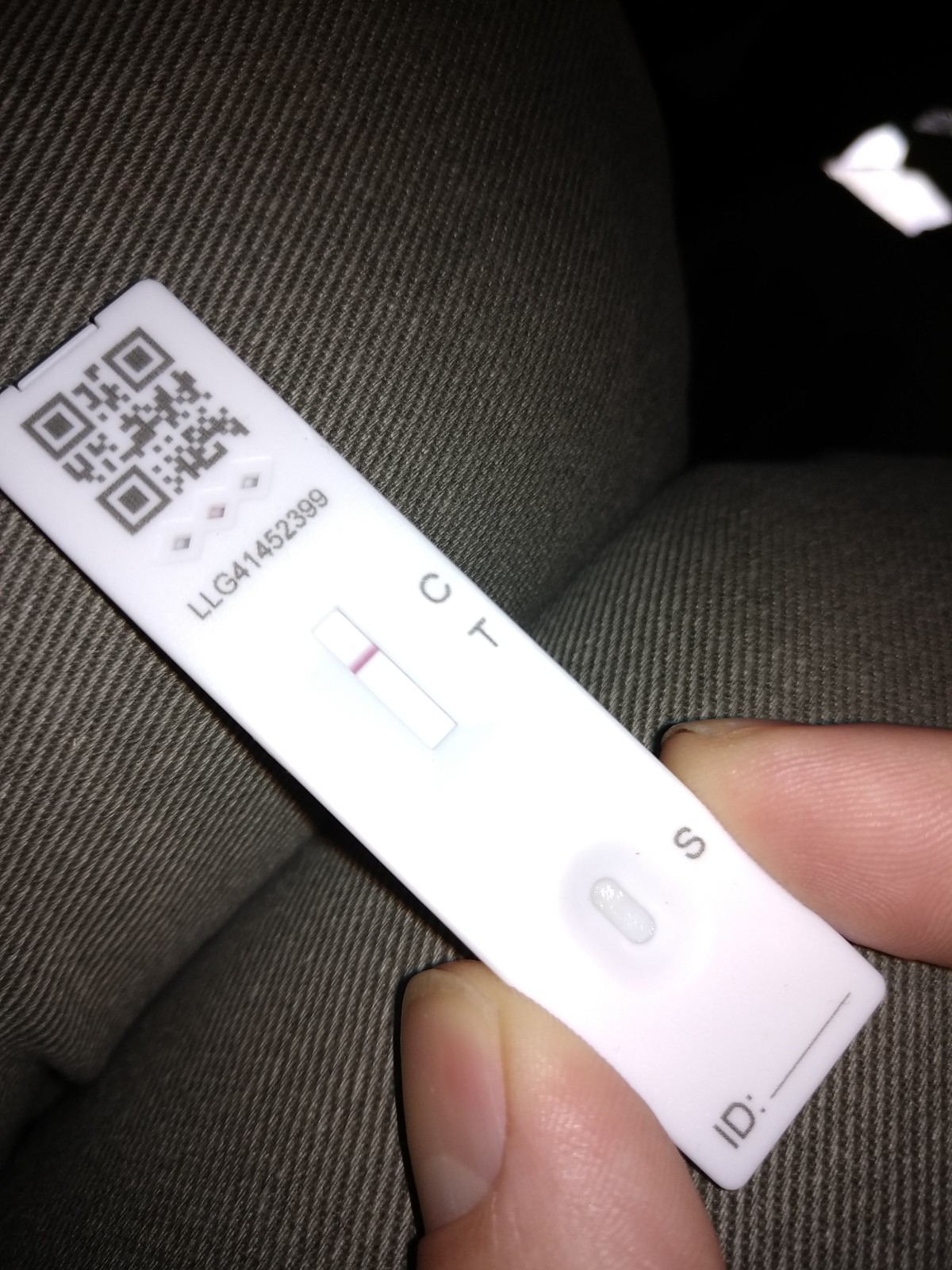In this close-up image, a hand is holding a white plastic test strip. The top of the strip features a prominent black QR code. Just below the QR code are three diamond-shaped indicators, which appear to function as lights or markers. Further down, there is a line of black text reading "LLG 41452399". Under this text, a large white rectangle is visible, with a red line running horizontally through it. Adjacent to the rectangle, there are letters indicating "C" above and "T" below, with the red line aligning with the "C". At the very bottom of the test strip, there is an oblong oval shape next to the letter "S", accompanied by the text "ID" and a blank line intended for user input. The background of the image shows a gray office chair, suggesting the setting is in a workspace or similar environment.